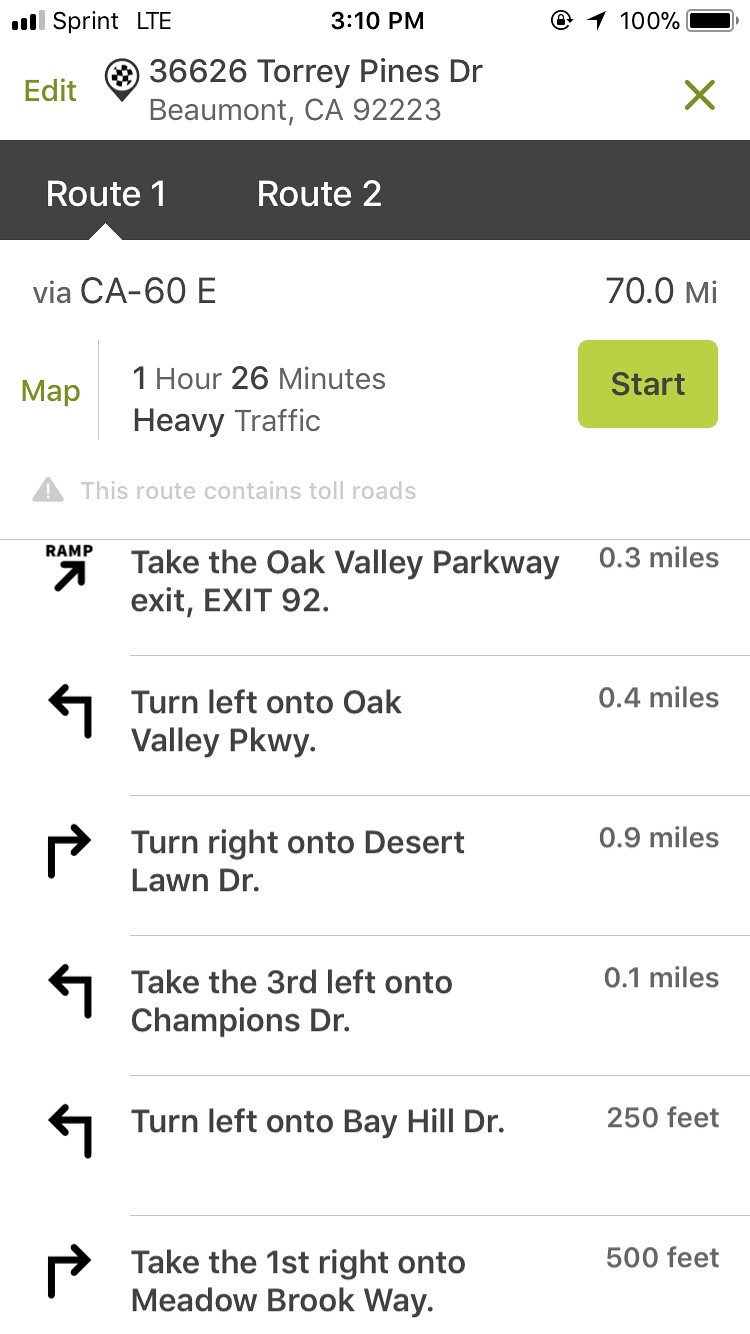This is a detailed screenshot of a GPS navigation interface displayed on a Sprint mobile phone, guiding the user to 36626 Torrey Pines Drive, Beaumont, CA 92223. The user has selected Route 1, which proceeds via California Highway 6 East. The interface indicates that the total distance is 70 miles, with an estimated travel time of 1 hour and 26 minutes in current heavy traffic conditions. Below, the screenshot provides a step-by-step breakdown of the directions:

1. Take the ramp onto California Highway 6 East.
2. Take exit 92 for Oak Valley Parkway.
3. Turn left onto Oak Valley Parkway.
4. Turn right onto Desert Lawn Drive.
5. Make the third left onto Champions Drive.
6. Turn left onto Bay Hill Drive.
7. Take the first right onto Meadowbrook Way.

The directions conclude at this final step.